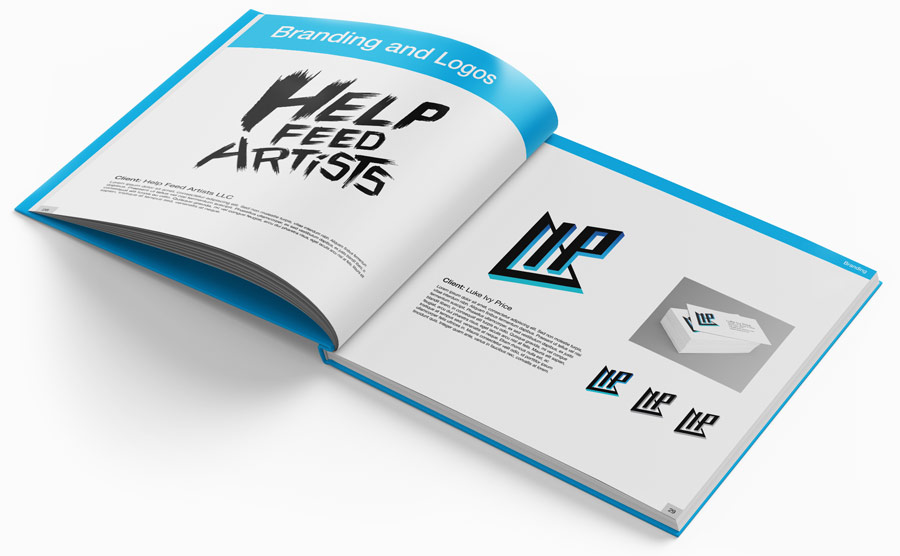The image depicts an open book positioned at a diagonal angle, starting from the top left corner to the bottom right on a blank, white surface. The book features predominantly light blue, black, and white hues. On the left-hand page, the header reads "Branding and Logos" in bold text, followed by the phrase "Help Feed Artists" in black and white, with additional smaller text beneath it. The right-hand page displays the initials "L-I-P," with the "L" crafted into a triangular shape. Also on the right page is a stack of three business cards bearing the same "L-I-P" logo. Below the logos and business cards, there is further descriptive text, though it is too small to discern clearly.